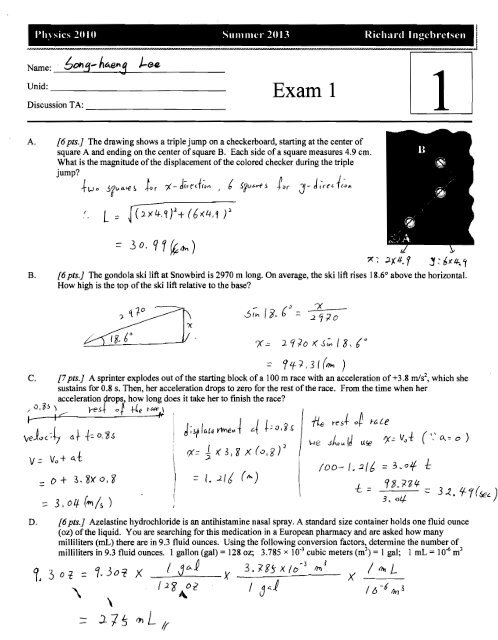This black and white scanned image depicts an examination paper labeled "Physics 2010, Summer 2013" authored by Richard Ingehretsen. At the top left corner, it lists "Name: Song-Hang Lee" and prominently displays "Exam 1" in black text. The exam paper features a series of mathematical problems and diagrams, including a triangle with specified angles and a shape resembling a side-laid ice cream cone. The layout includes columns of text and equations too small to decipher clearly. Various sections are denoted by the letters A, B, C, and D, each containing problem statements or solutions, along with handwritten responses and calculations throughout.